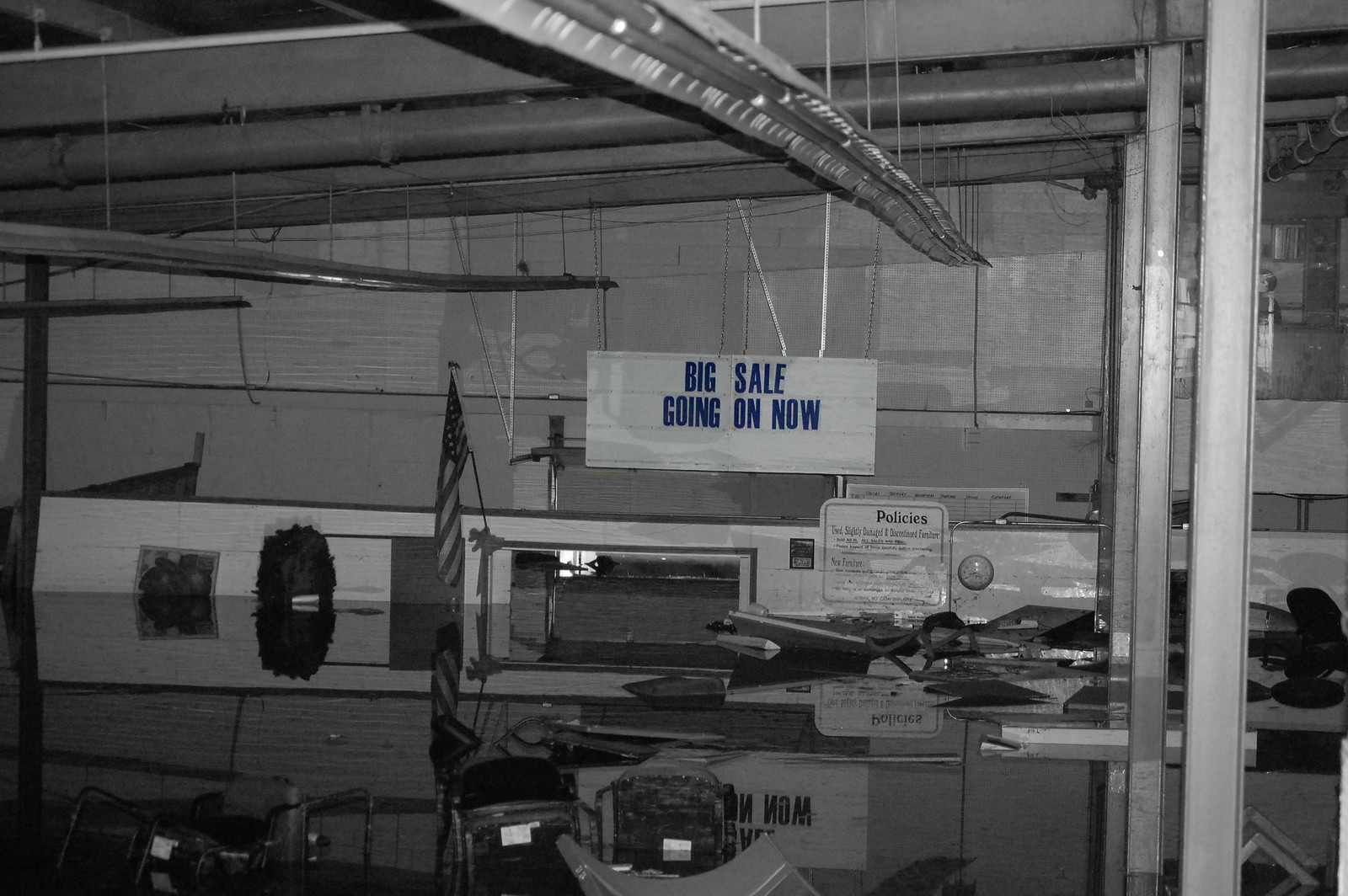The image depicts an indoor scene with a high ceiling featuring horizontal gray pipes running left to right. There are chains connected to the ceiling pillars, mounting a banner in the center. This central white banner has large black text printed on it and features an American flag in its bottom left corner. The space appears to be an old, possibly abandoned store with a chaotic layout and a reflective surface on the floor that suggests flooding, as various items, including some submerged vehicles and black metal desks, float in the water. White metal pillars stand to the right of the image, supporting the structure. The overall scene is in black and white, enhanced with some color, primarily in the central banner and flag. The store has a desolate and tragic atmosphere, emphasized by the mess and the still water flooding the space.